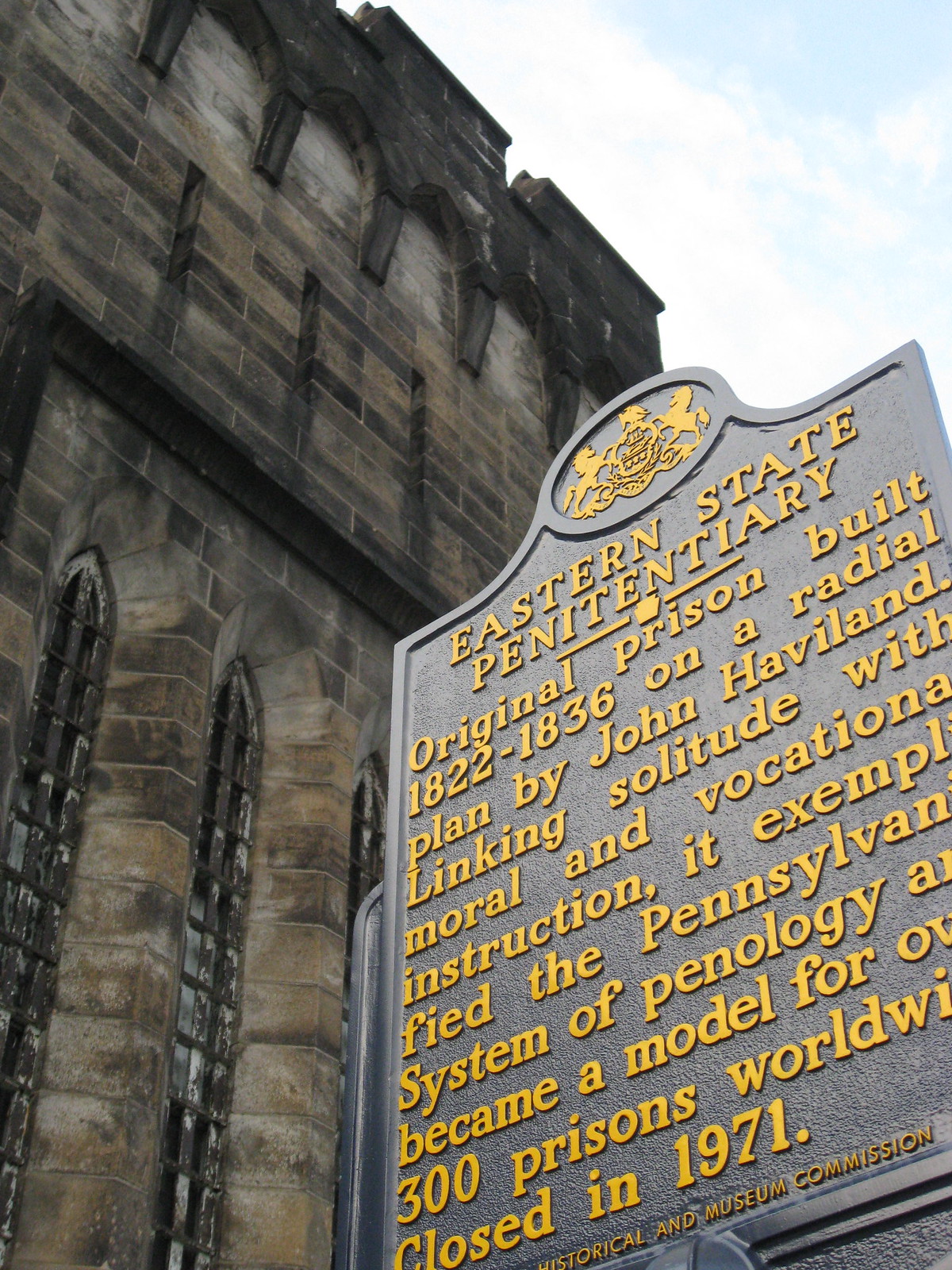The photograph captures an elegant metal plaque against a dark blue background, inscribed with gold text. The sign reads: "Eastern State Penitentiary. Original prison built 1822 to 1836 on a radial plan by John Haviland, linking solitude with moral and vocational instruction. It exemplified the Pennsylvania system of penology and became a model for over 300 prisons worldwide. Closed in 1971." At the bottom, in smaller letters, it mentions the Historical and Museum Commission. To the right of the plaque stands a formidable, weathered stone building that resembles a fort or perhaps a cathedral due to its tall, arched windows. The structure is old and covered with signs of age, like mold and mildew, adding to its imposing presence. The vantage point of the photo is slightly below the sign, allowing for a glimpse of the blue sky with scattered white clouds in the upper right corner.